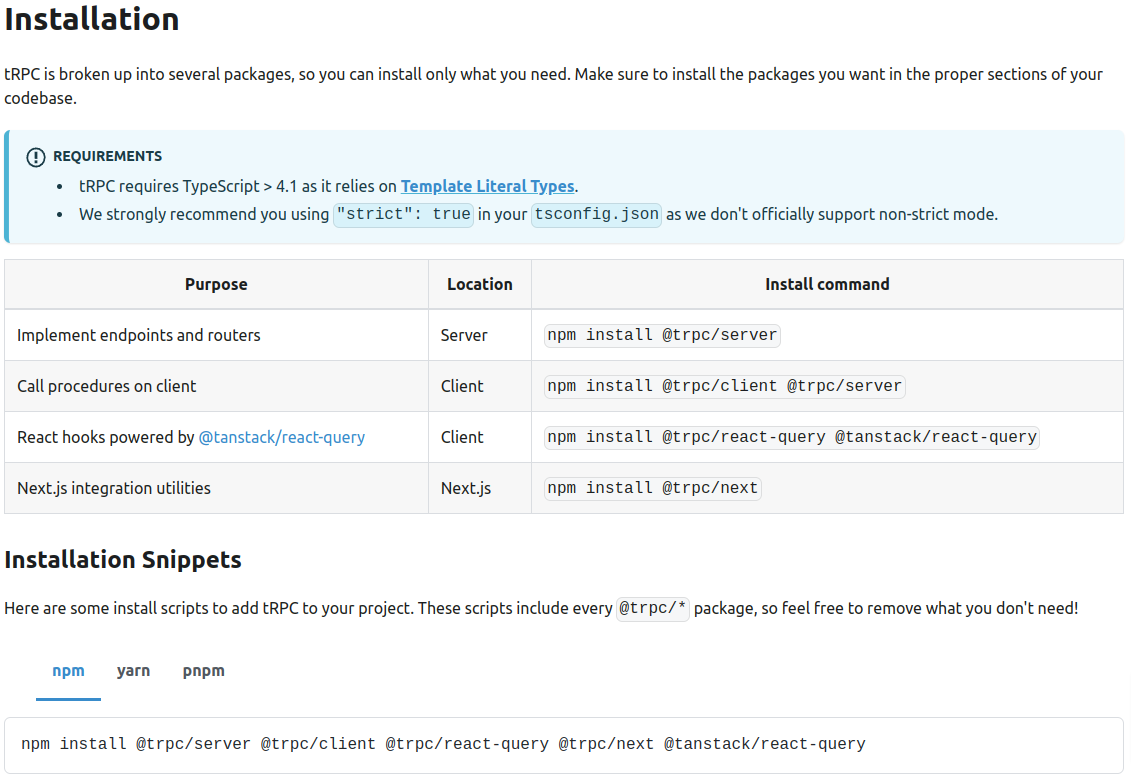Screenshot of TRPC Installation Instructions

The screenshot provides detailed installation instructions for TRPC, ensuring the process is broken down into modular packages so developers can install only what they need. TRPC is noted for its necessity to integrate with TypeScript, indicated as "TypeScript" with a capital "T" and "S." The screenshot emphasizes that TRPC requires TypeScript version 4.1 or higher due to its reliance on template literal types, mentioning this feature with a blue hyperlink for further reference.

Additionally, the screenshot strongly recommends setting the `strict` option to `true` in your `tsconfig.json` file, as non-strict mode is not officially supported by TRPC.

A table is included to assist users in understanding the purpose, location, and corresponding installation commands for the different TRPC packages:

- **Purpose**: Implement endpoints and routers
  - **Location**: Server
  - **Install Command**: `npm install @trpc/server`

- **Purpose**: Call procedures on the client
  - **Location**: Client
  - **Install Command**: `npm install @trpc/client @trpc/server`